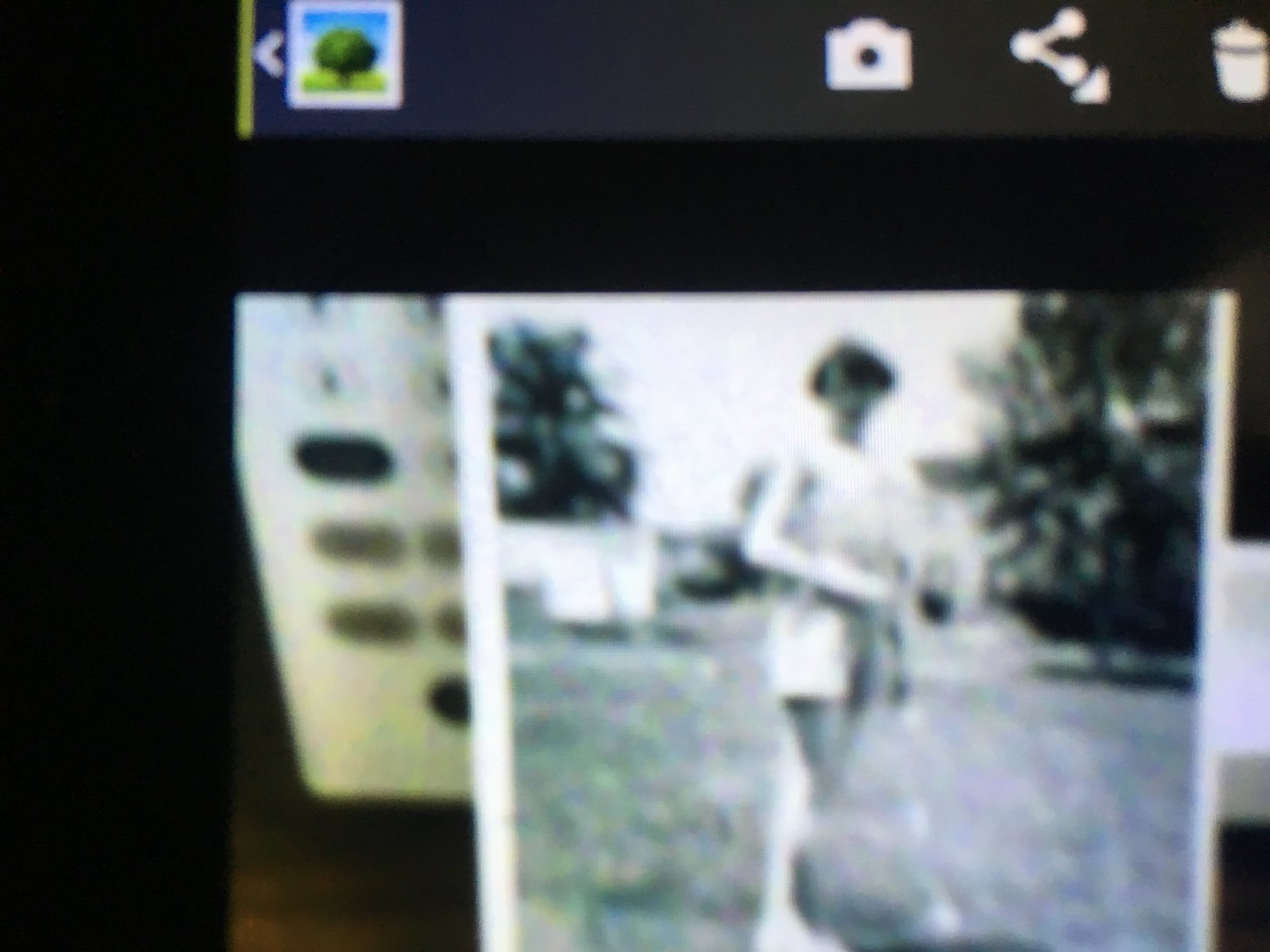A grainy black-and-white photograph from what appears to be the 1950s or 1960s captures the image of a Caucasian woman standing outdoors. She is dressed in a sleeveless, short top paired with shorts, and has very short black hair. The woman’s bare legs are visible, and she holds an indistinct object, possibly a stick, cane, or club, in her left hand. The setting features trees and a house in the background to the right, with grass visible to the left, suggesting she may be standing in a driveway. 

The photo occupies the middle to far right portion of the frame and is bordered in black. Above the photograph, elements of a computer screen are visible, including a small box depicting a green tree against a blue sky, a white camera emblem, a search bar, and a delete button on the right side. The overall image is quite blurry, adding a sense of mystery and nostalgia to the scene.